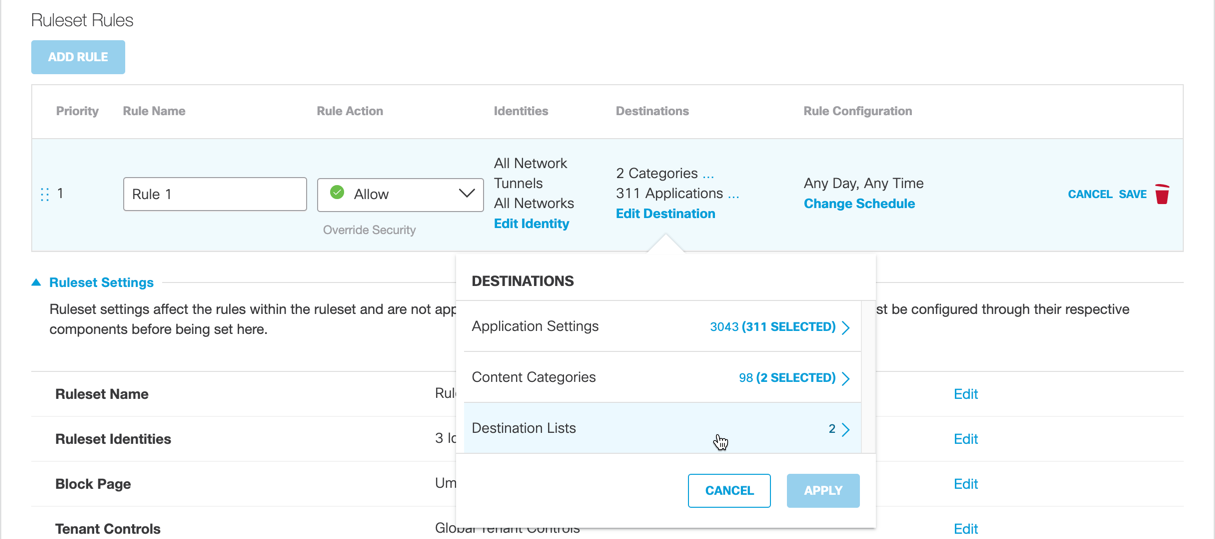This image depicts a web interface predominantly styled in light colors. The top left corner features the label "Reset Rules." Below this, there is a light blue button labeled "Add Rule." Spanning across the webpage is a white box containing column headings: "Priority," "Rule Name," "Rule Action," "Identities," "Destinations," and "Rule Configuration."

Beneath this section is another light blue box, which contains two white boxes. One of these boxes is labeled "Rule 1," and the other is labeled "Allow." The "Allow" button is marked with a small green circle and a check mark. Additional text within this section includes "All Network," "Tunnels," "All Network," and "Edit Identity" in blue text. It also categorizes information under "311 Applications," "Edit Destination," and "Any Day, Any Time," alongside a prompt to "Change Schedule."

Towards the bottom, options for cancelling or saving changes are presented, alongside a red trash can icon. Further down, there's a section titled "Rule Set Settings," containing a description that clarifies these settings influence rules within the rule set and are not app components until configured here. The section lists items such as "Rule Set Name," "Rule Set Identities," "Block Page," and "Tenant Controls."

Overlaying the main interface is a pop-up window labeled "Destinations." Within this pop-up, there are sections for "Application Settings," "Content Categories," "Destination Lists," as well as numerical indicators running down the right side of the page. The pop-up also provides "Cancel" and "Apply" buttons, with four "Edit" buttons on the left side for modifying the listed information.